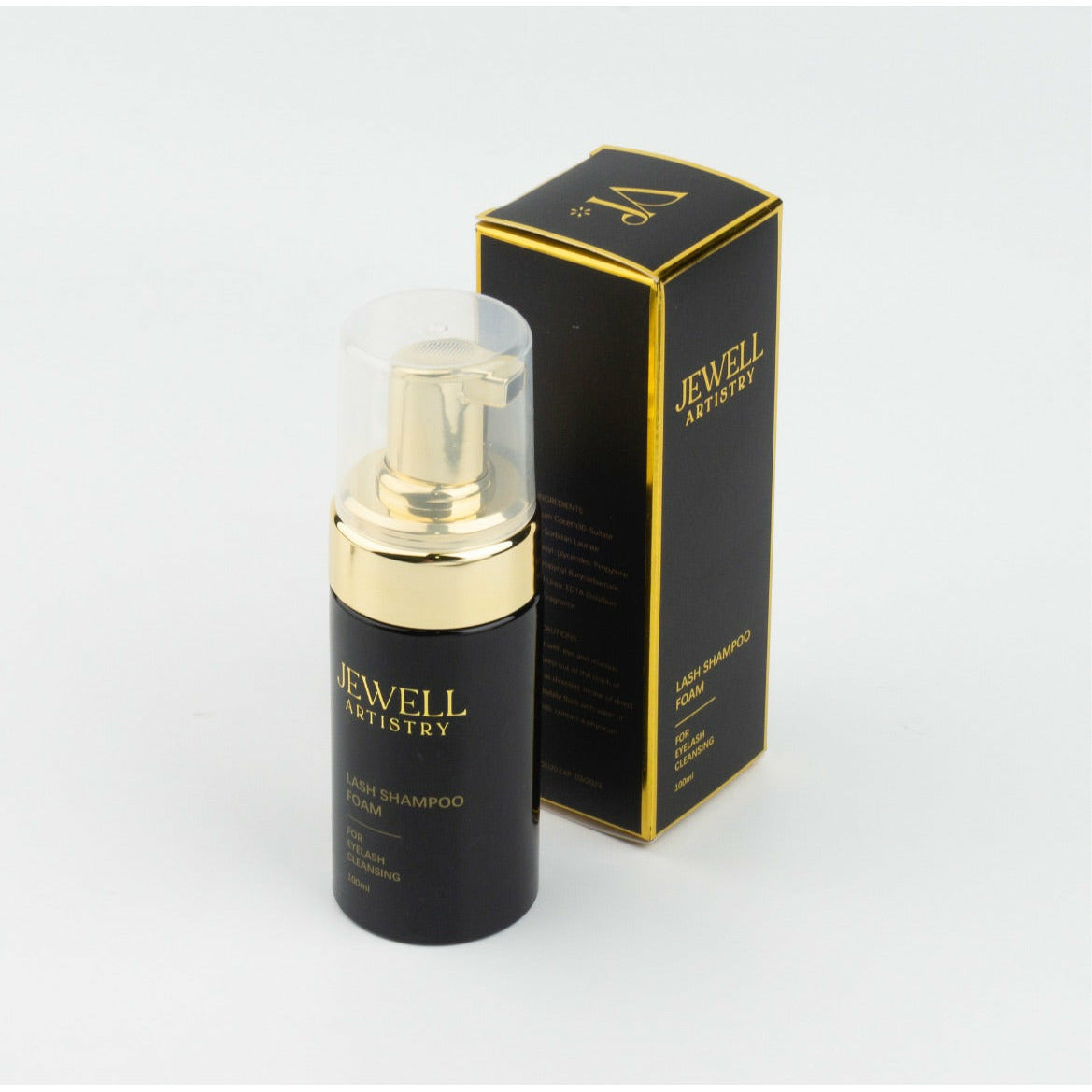The image portrays a product setup showcasing the Jewel Artistry Lash Shampoo Foam, photographed against a light bluish-gray background in a square format. At the forefront is a cylindrical plastic bottle, elegantly designed with a clear cap and a gold pump dispenser. The bottle features a black base adorned with a gold metallic label that reads "JEWEL ARTISTRY" and "Lash Shampoo Foam." Positioned just behind the bottle is the product's packaging—a black, rectangular box accented with gold trim. The box is slightly angled, displaying both its front and a glimpse of the back, prominently featuring the brand name "Jewel Artistry" in gold at the top and "For Eyelash Cleansing" below. This meticulous composition highlights the sophisticated and luxurious aesthetic of the lash shampoo product.